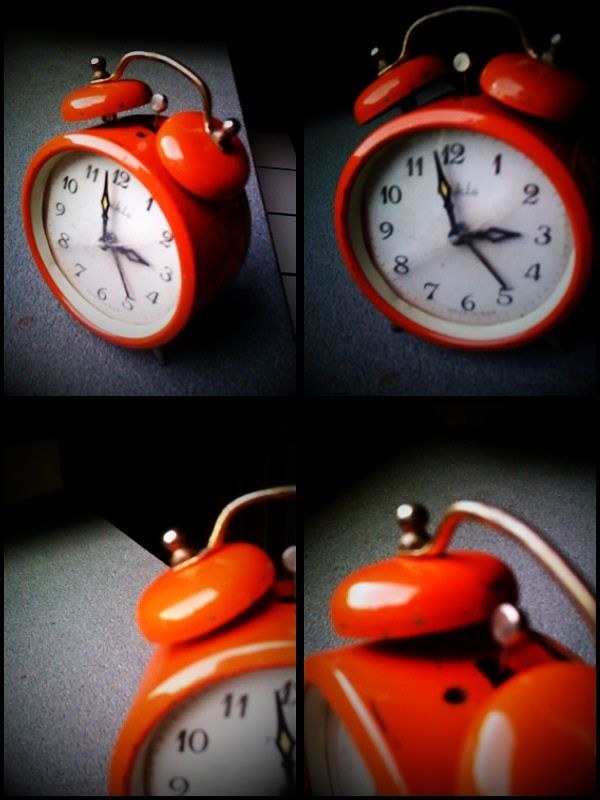A 2x2 grid displays four distinct angles of a vintage red alarm clock, emphasizing its timeless design. The clock features a classic circular analog face with bold black numerals and sleek black hands that enhance its readability. Atop the clock sit two gleaming metal bells, connected by a miniature pendulum-like ringer poised to chime. The meticulously crafted antique piece exudes charm, capturing the essence of a bygone era with its vibrant red hue and intricate details.